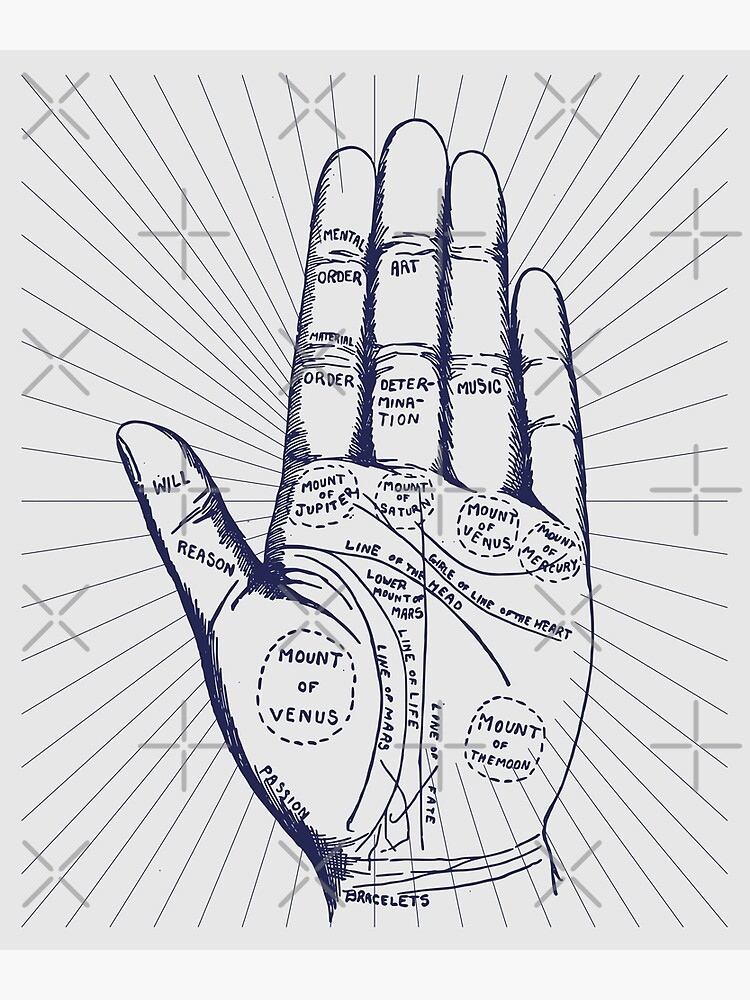The black ink drawing features a detailed depiction of a left hand with the palm facing outward. The palm is inscribed with various labels and lines, with terminology specific to palmistry. On the thumb, the words "Will" and "Reason" are visible. The index finger bears the labels "Mental Order" and "Material Order," while the middle finger reads "Art" and "Determination." The ring finger is marked with "Music." Each of the mounts within the palm is designated: "Mount of Venus," "Mount of Jupiter," "Mount of Saturn," and "Mount of Mercury," while the bottom right corner of the palm features "Mount of the Moon." Additionally, the wrist area contains the word "Bracelets."

Surrounding the hand are numerous lines radiating outward, converging towards the palm, creating a starburst effect. Interspersed among these lines are star and cross-like symbols, adding to the intricate, celestial theme. Some areas of the palm are circled or have lines drawn through them, emphasizing the palm's detailed and mystical attributes.